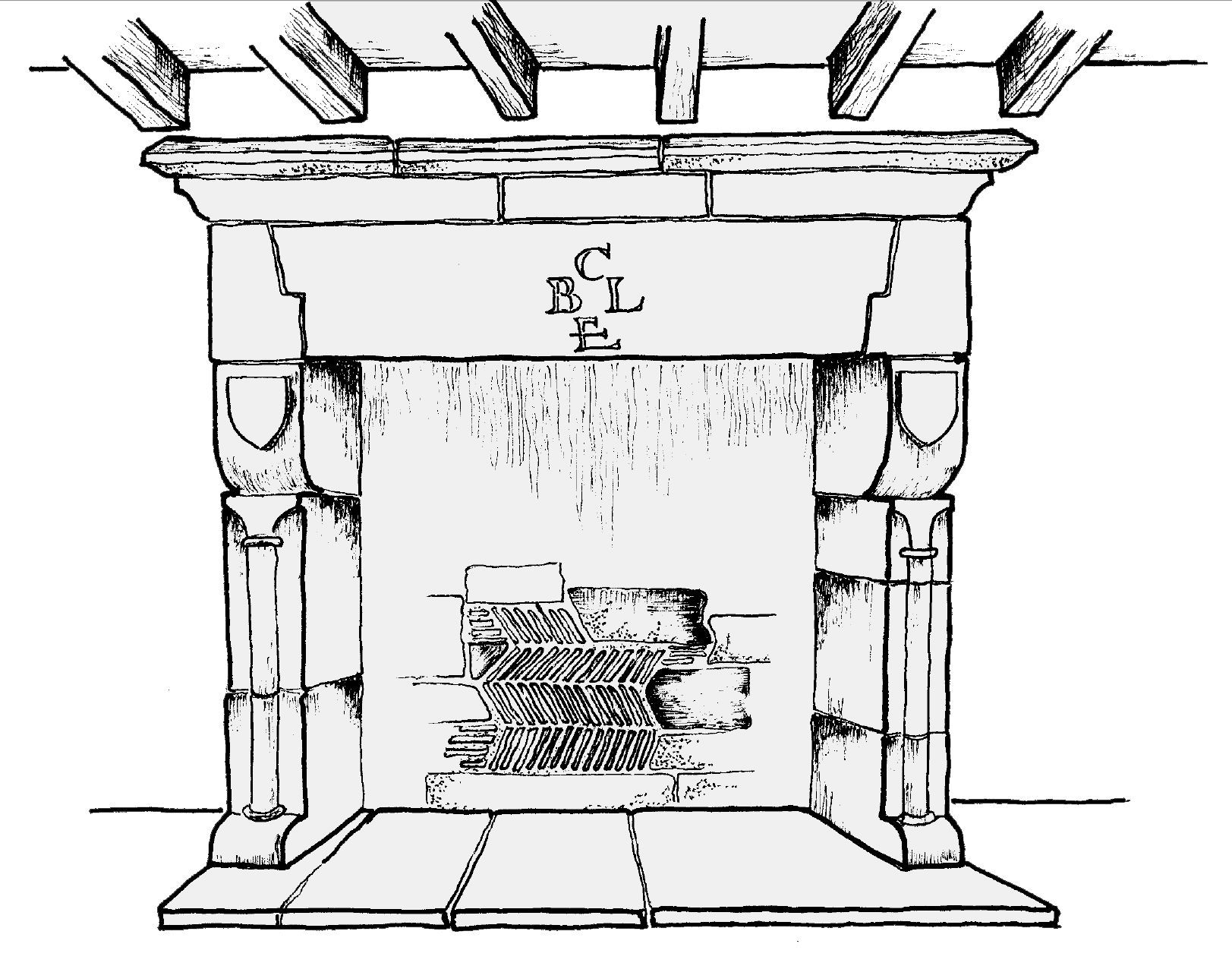This is a black and white drawing of a centered, floor-to-ceiling fireplace, rendered with minimal details and grayscale shading. The fireplace is constructed of gray brick or concrete and features two prominent columns on each side. Inside, there are metal grates and rectangular wooden logs, with no fire currently burning. At the very top of the image, some ceiling rafters or boards are visible, suggesting the room's structure. Above the fireplace, there are letters engraved in a circular pattern that read "C, B, L, E" arranged in a clockwise manner. Additionally, there appear to be two coat-of-arms-style emblems flanking the sides of the fireplace, contributing to its modestly ornate design. The overall scene suggests a homely or possibly hotel-like setting.